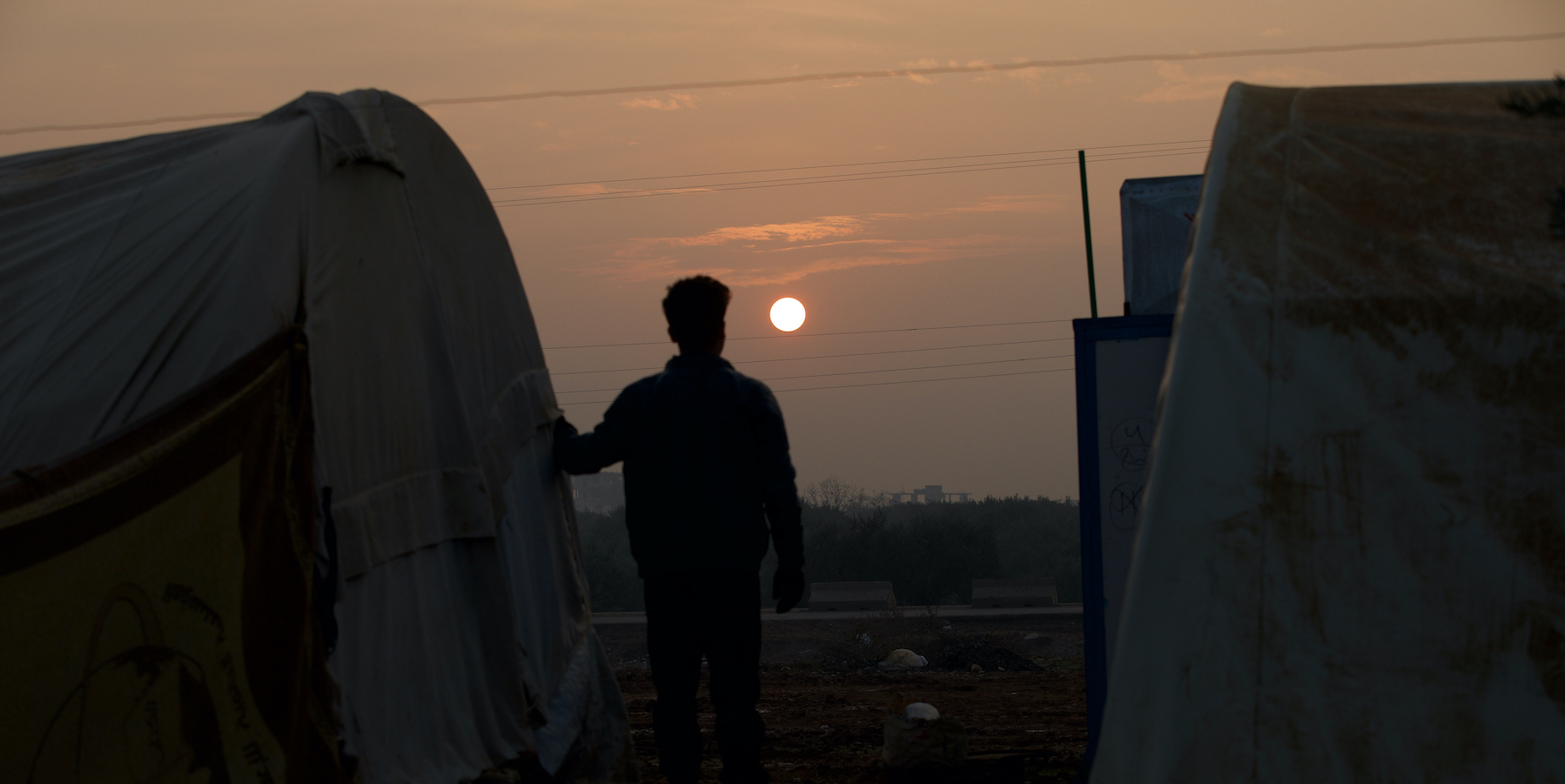This photograph captures a night-time scene with a blurry yet compelling atmosphere. Dominating the center is the outline of a man, his hair discernible as it stands atop his head. He is resting his left arm on what appears to be a tent, though the darkness obscures precise details. The scene suggests it is a makeshift village, possibly a refugee tent city, given the tents depicted on the left and right sides of the image.

The sky above is a gradient of colors, transitioning from gray clouds to a subtle pink hue, indicative of either sunrise or sunset. The man is staring at a perfectly round, yellow orb in the sky, most likely the setting sun. The lower half of the image is shrouded in darkness, making it difficult to distinguish objects, but hints of trash on the ground and power lines overhead are faintly visible. There is also a flag on the left side of the photograph, adorned with a yellow and red symbol, though the text is indiscernible.

The tents are white, contrasted against the primarily brown dirt of the ground. The overall composition emphasizes the solitary figure of the man against the backdrop of the setting sun, enveloped by the stark and somber ambiance of the tent village.